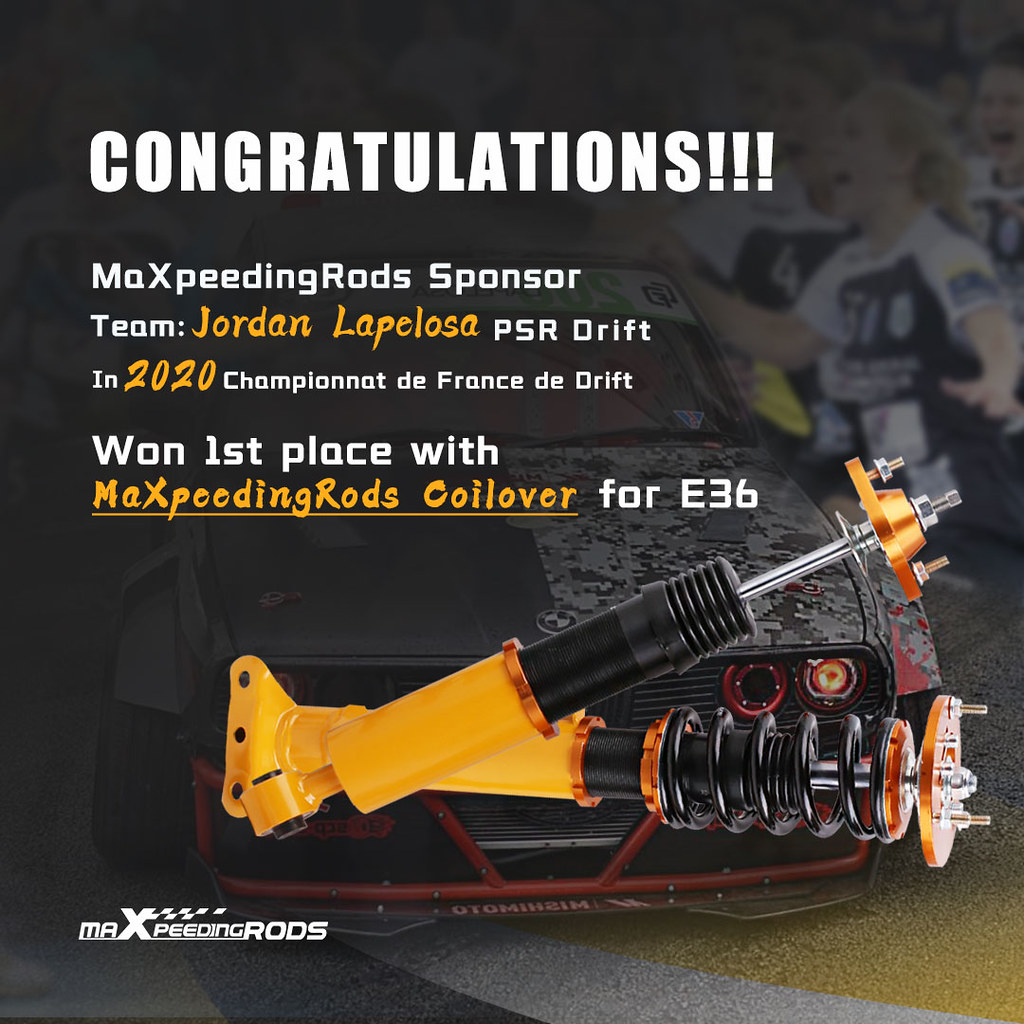The square poster features a predominantly black background with the word "Congratulations" boldly displayed at the top in white letters. The poster is both a celebratory message and an advertisement. It announces that Team Jordan Lapalosa PSR Drift secured the "Champion de France de Drift" title in 2020, with a reference to their winning first place using Maxpeedingrods Coilovers for an E36.

Visual elements on the poster include a black BMW adorned with gray camo on one side and dark red highlights, including a dark red headlight and a yellow headlight. The bottom of the image showcases two car coilovers, which are yellow at the base and feature screws at the top, indicating that these are the Maxpeedingrods Coilovers mentioned.

The text is layered over faint images of celebrating crowds and the race car, reinforcing the dual nature of the poster as both a proclamation of victory and an advertisement. The bottom of the poster prominently shows the Maxpeedingrods logo, reinforcing this sponsorship.